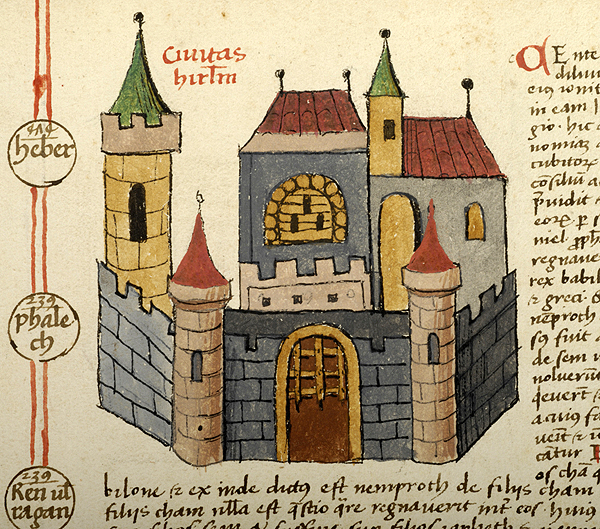The image is a vintage, color illustration on an older, beige, off-white paper with a dingy appearance. The centerpiece is a colorful castle with multiple towers, rendered in flat sections of yellow, blue, red, gold, green, and orange, and featuring brick-red, corrugated-style roofs. Above the castle is a headline in a different language, accompanied by more text underneath the castle in a similar medieval script. On the right side, a prominent paragraph is written in an old penmanship style, also in a foreign language. To the right of a green tower, illegible orange text adds to the aura of antiquity. On the left side, two vertical orange lines connect three circles spaced apart vertically—top, middle, and bottom—each containing black script writing in a foreign language. The illustration is in landscape orientation and exudes a vintage charm through its detailed and colorful depiction.